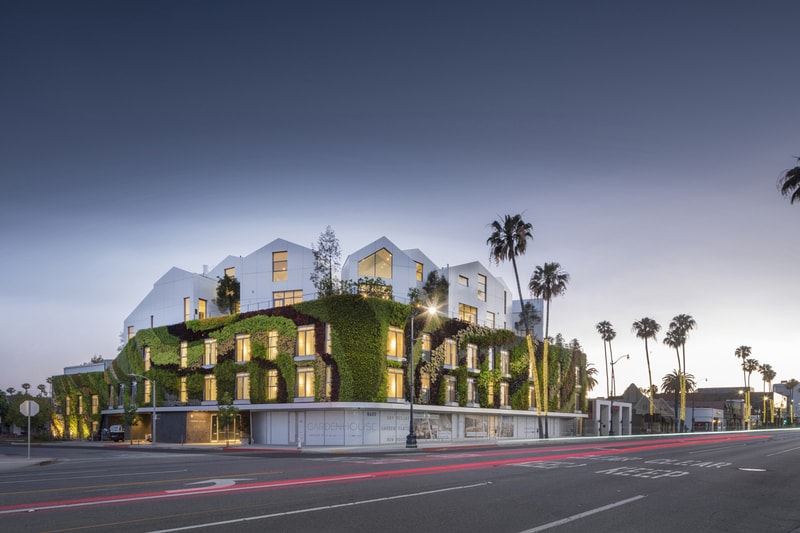This image, captured during daylight, depicts a striking city intersection dominated by a prominent, multi-story residential building, possibly apartments or condos. The sky above presents a dramatic gradient, from an almost black hue at the top to a lighter, hazy white near the bottom. The building's lower levels, constructed primarily from glass and metal, contrast with the second and third stories, where the facade is adorned with an eclectic mix of green, black, brown, and yellow vines, giving it an artistic and vibrant appearance. This plant-covered section creates a textured, living artwork that stands out against the building's mostly white exterior. The upper floors, or possibly adjacent structures, feature distinctive triangular shapes on top of square forms. The intersection itself is surrounded by numerous palm trees, and large roads intersect the scene, running from the bottom left to the top right, with a turn to the left, indicating it’s a corner block area. Despite the urban setting, there are no visible cars on the streets, giving the photograph a serene, almost surreal quality with the yellow lights emanating softly from the building, suggesting twilight.